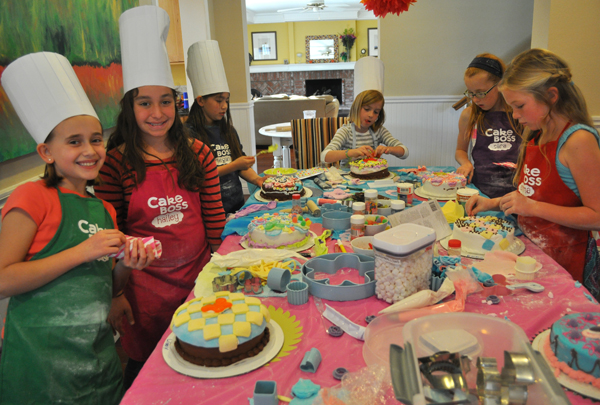In this vibrant, indoor image, a group of six elementary school-aged girls are gathered around a rectangular table draped in a pink tablecloth, celebrating what appears to be a birthday party. The scene is filled with the bustling activity of cake decorating. Each girl is clad in a colorful "Cake Boss" apron, displaying hues of green, red, purple, and blue, with individual names embroidered on them. Four of the girls are also wearing tall white chef's hats, adding an extra touch of authenticity to their roles as budding cake decorators. The atmosphere suggests a summertime setting, as many of the girls wear tank tops and t-shirts that are slightly sun-kissed.

The table is a cake decorator's paradise, laden with an impressive array of cake-making tools, utensils, and toppings, including chocolate chips, marshmallows, sprinkles, and various types of icing. Each girl has a round cake in front of her, with some cakes nearly completed and others still in the decorating process. The girls in the front beam at the camera with big smiles, clearly proud of their creations, while the others are engrossed in adding the finishing touches to their cakes. The background features an open doorway leading to a family room, suggesting the cozy intimacy of a home setting. The overall scene is a delightful burst of colors and creativity, embodying the joy and excitement of a special celebration.